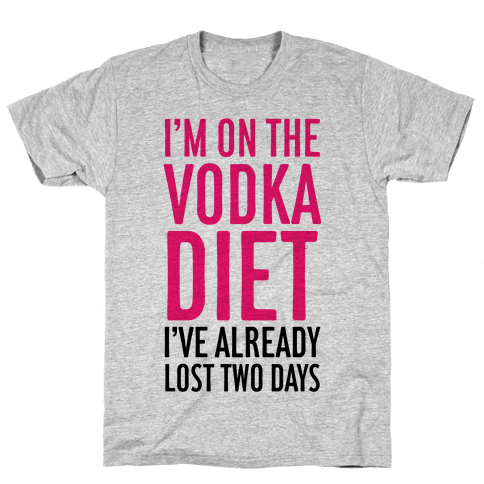The image showcases a heather gray short-sleeved t-shirt laid out on a white background. The t-shirt is slightly wrinkled, suggesting it was taken from the laundry and half-heartedly smoothed out. The shirt features a bold, humorous message in large, capital letters. The text reads: "I'm on the Vodka Diet" in a dark pink or magenta sans-serif font, with the word "Diet" being the largest. Beneath this, in smaller black text, is the phrase: "I've already lost two days." This punchline humorously intimates a loss of time, presumably from heavy drinking. The shirt appears to have no visible size or tag, possibly indicating the tag has been removed or is sewn inside.